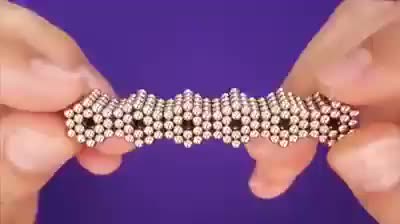In this horizontal, rectangular image, the background features a solid blue-purple hue. On the far left and right edges, two hands emerge, each set of fingers grasping a central metallic object. The fingers on the left side only reveal the fingernails and the very beginnings of the fingers, while the fingers on the right side expose a bit more, though not reaching the knuckles. The object being held is an intricately worked piece of metal composed of small, interconnected components, reminiscent of metallic beads or magnets. These components are arranged in a strip of six hexagonal prisms, each with hollow centers resembling the structure of metallic watch bands. The hands are fair to tan in color, and they hold the metallic piece straight, stretching it horizontally across the vibrant, monochromatic background.